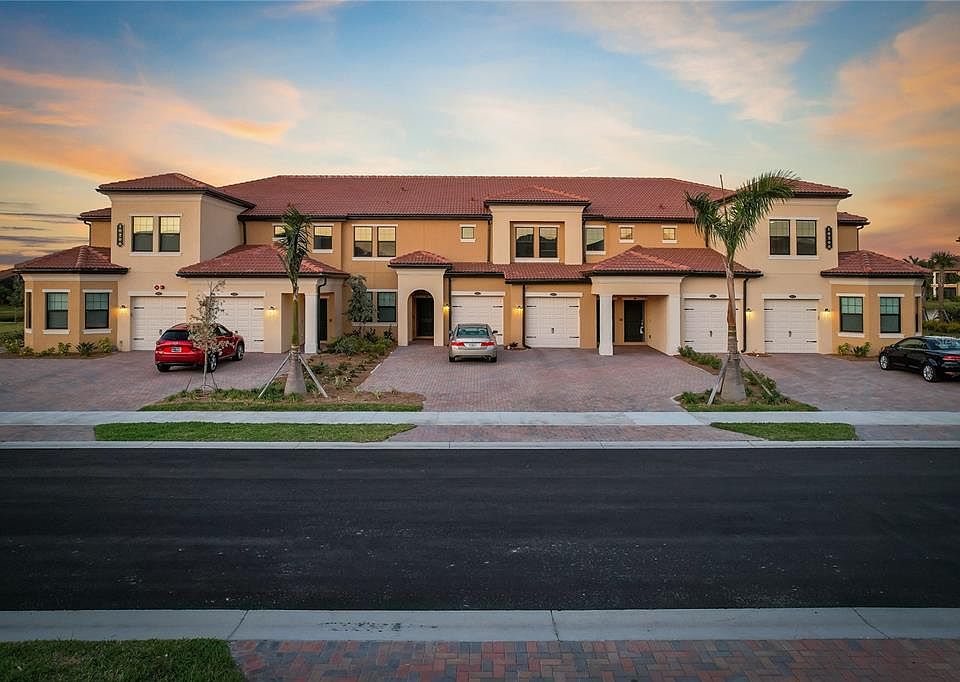This image features a multi-family dwelling, most likely townhouse apartments or condos, situated in a warm climate, potentially the western United States such as Arizona. The building is a two-story structure with a camel-colored or sandy brown facade complemented by cream or beige accents. Its roof is a reddish maroon, possibly tile, emphasized by the rounded turret-style outcroppings on either end of the building, each featuring windows that might serve as breakfast nooks.

The frontage presents three distinct homes, each with an arched doorway, two single-car white garage doors, and several windows, including 12 larger windows and numerous smaller ones on the second floor. The garage doors and front entrances are symmetrically laid out along the well-maintained asphalt road, which features newly laid grass islands and a fresh sidewalk.

In front of the homes, there are three cars parked: a red car on the left, a silver sedan in the middle, and a dark blue or black car on the right. Additionally, two tropical-looking palm trees with slender trunks stand near the sidewalk, contributing to the warm climate aesthetic. The sky above is vibrant blue, tinged with pink hues, suggesting the photo was taken during sunrise or sunset.